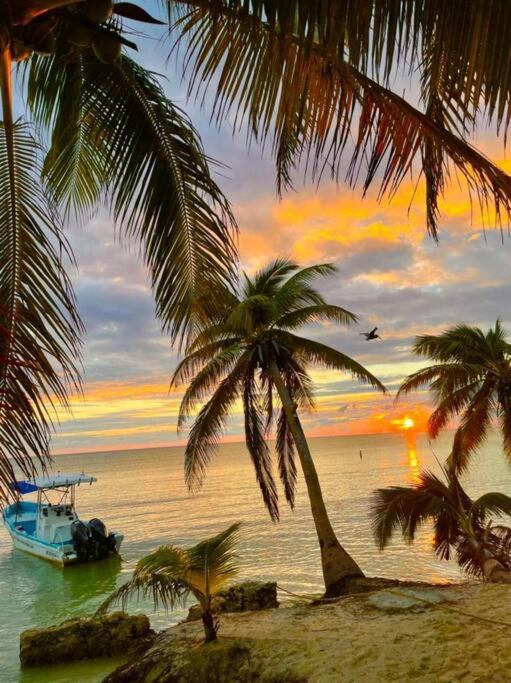The image portrays a picturesque tropical island scene during sunset. Dominating the foreground are several palm trees, with their fronds gracefully arching over the frame, both from above and along the sandy shore, where a few smaller palm trees stand near some protruding rocks. The ocean stretches out calm and nearly waveless, tinted with a greenish hue, reflecting the golden-pink glow of the setting sun. The sky is a dramatic blend of blue, gray, and cloud-streaked shades of yellow, orange, and pink, casting a warm, mottled light across the scene. Anchored a short distance from the beach is a small fishing boat, identifiable by its twin outboard motors, blue canopy, and light blue interior set against a white exterior. The serene and tranquil scene is accentuated by a lone black bird flying in the distance, adding a touch of life to this idyllic tropical vista.